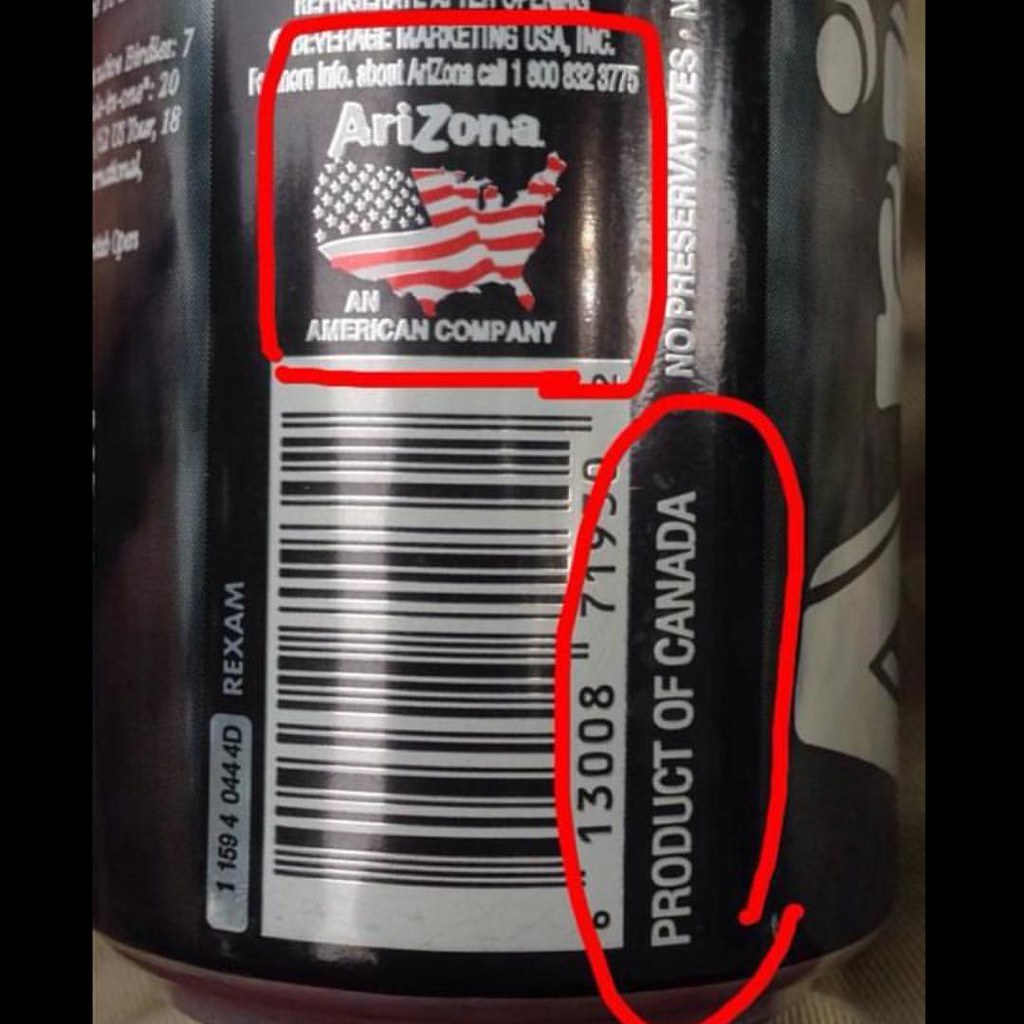An extremely close-up image of a beverage container vividly showcases specific details highlighted with digital annotations. To the left, a red digital pen has circled the barcode with adjacent white text stating "Product of Canada." Higher up, near the top of the image, an orange virtual marker underscores the Arizona Tea logo alongside an address indicating where the drink is made. This segment also includes an illustration of the continental United States overlaid with an American flag and the phrase "An American company." These highlighted sections emphasize key origin details of the beverage.